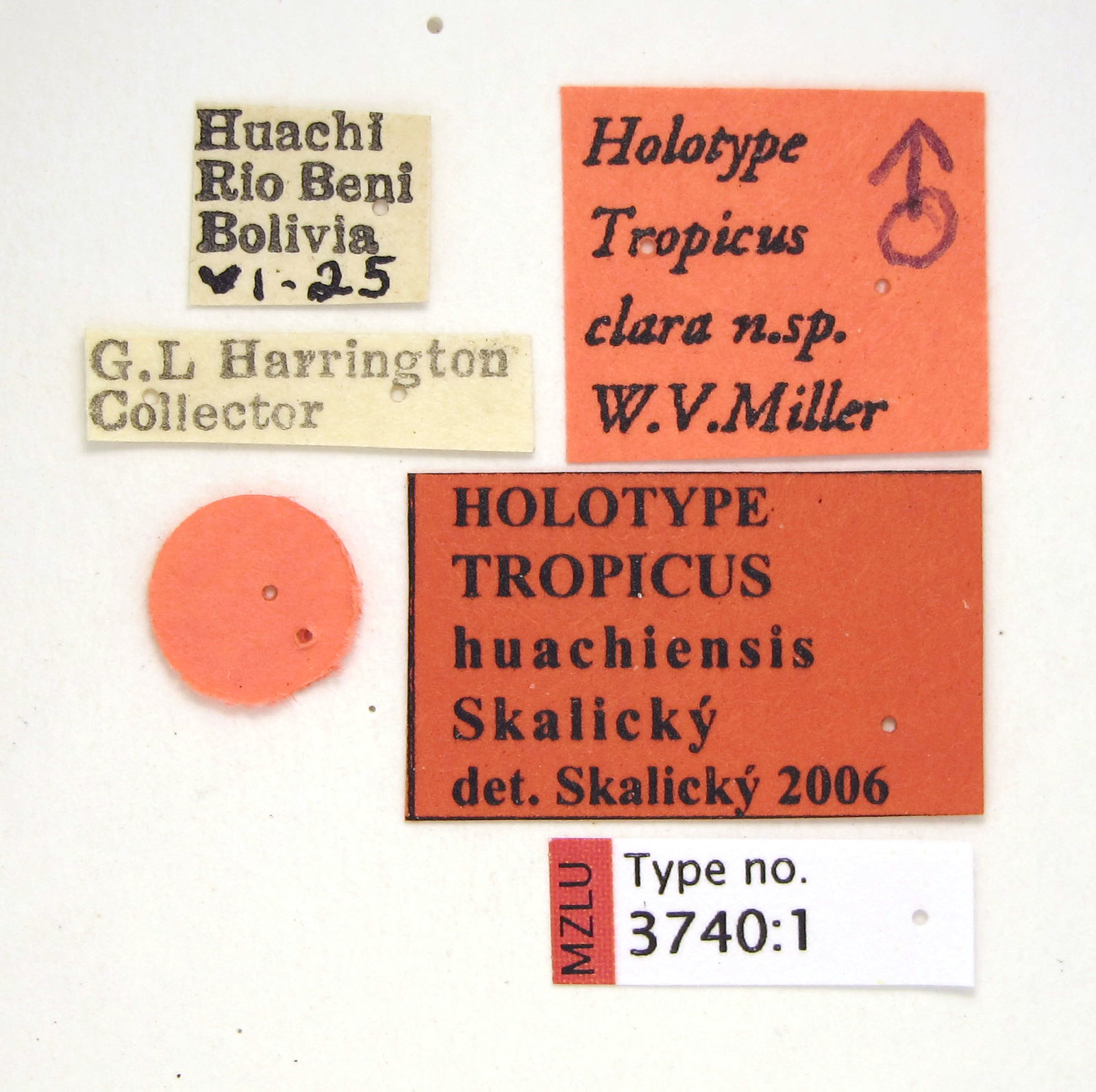The image depicts a wall adorned with various posters, stickers, and writings, none of which are in English. The display includes six distinct items: three orange posters positioned in the top right and middle right areas, with an orange circle on the left. Below the orange posters, there's a red and white item resembling a ticket. In the top left corner, there's a yellow sticker and a yellow piece that resembles a newspaper headline. One square sticker, red in color, reads "Holotype, Tropicus, Clara, NSP, WV, Miller," accompanied by a male gender symbol pointing upwards. Another rectangular piece notes "GL Harrington Collector," while a second rectangular piece reads "Holotype, Tropicus, Hugo Exciensis, Skaliki Dead Skaliki 2006." One item, marked with a heart and "1-25," further adds to the eclectic mix of visual elements.